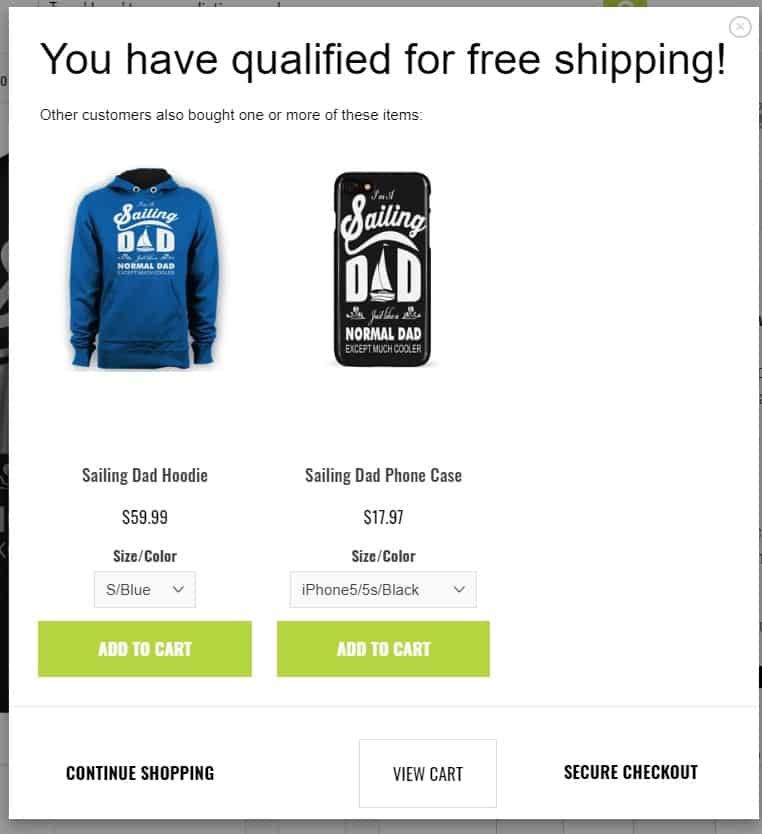Screenshot from a clothing e-commerce website featuring a shopping cart:

**Headline**: "You have qualified for free shipping"

**Banner**: "Other customers also bought one or more of these items"

**Product 1**: A vibrant blue hoodie with the text "Sailing Dad," where the letter 'A' is creatively designed as a sailboat. Priced at $59.99, the hoodie is available in various sizes and colors. The displayed option is Small in blue. There is a prominent green "Add to Cart" button next to the product details.

**Product 2**: An iPhone case featuring the text "Sailing Dad - normal dad on the back" specifically designed for the iPhone 5/5S in black. Priced at $17.97, this case also offers size and color variations. The option displayed is Black for the iPhone 5/5S. Similar to the hoodie, there is a green "Add to Cart" button next to this item.

**Navigation Buttons at the Bottom**: Options to "Continue Shopping," "View Cart," or proceed to "Secure Checkout" are available, allowing for easy navigation and purchase completion.

This detailed caption captures the essence of the shopping cart interface, including product descriptions, pricing, and available actions for the user.